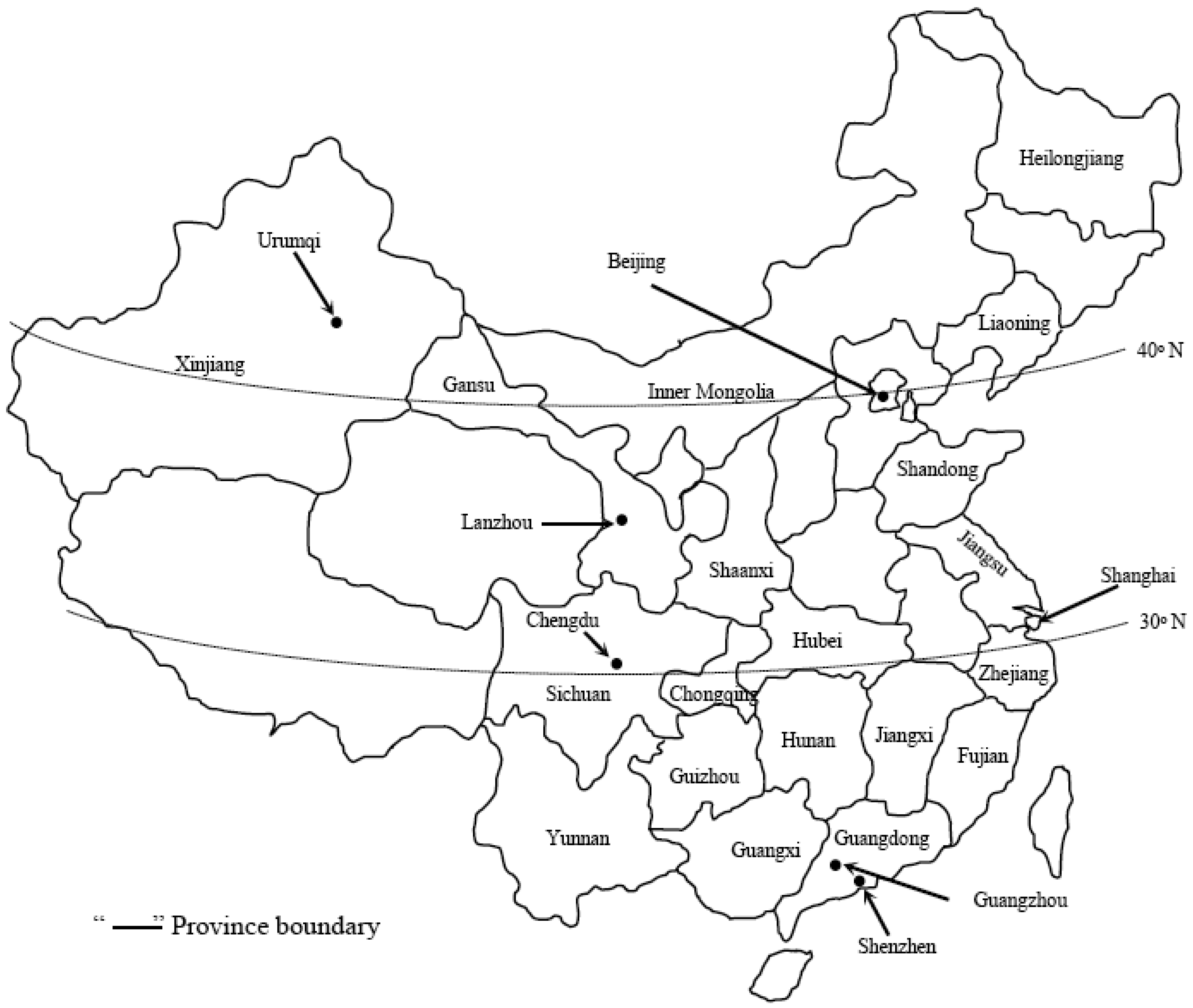This black-and-white map, likely hand-drawn with a black marker on a white surface, depicts the country of China with a unique and detailed outline. Each of the numerous provinces within China is labeled with names, such as Beijing, Hunan, Shanghai, Xinjiang, and Hubei, among others. The map includes province boundaries indicated by lines leading to dots. Additionally, horizontal lines marking the degrees of latitude, including 30 degrees north and 40 degrees north, are present, providing a geographical frame of reference. Simplistic in design, devoid of topographical features, the map's clean, modern appearance effectively focuses on the borders and names of various regions.